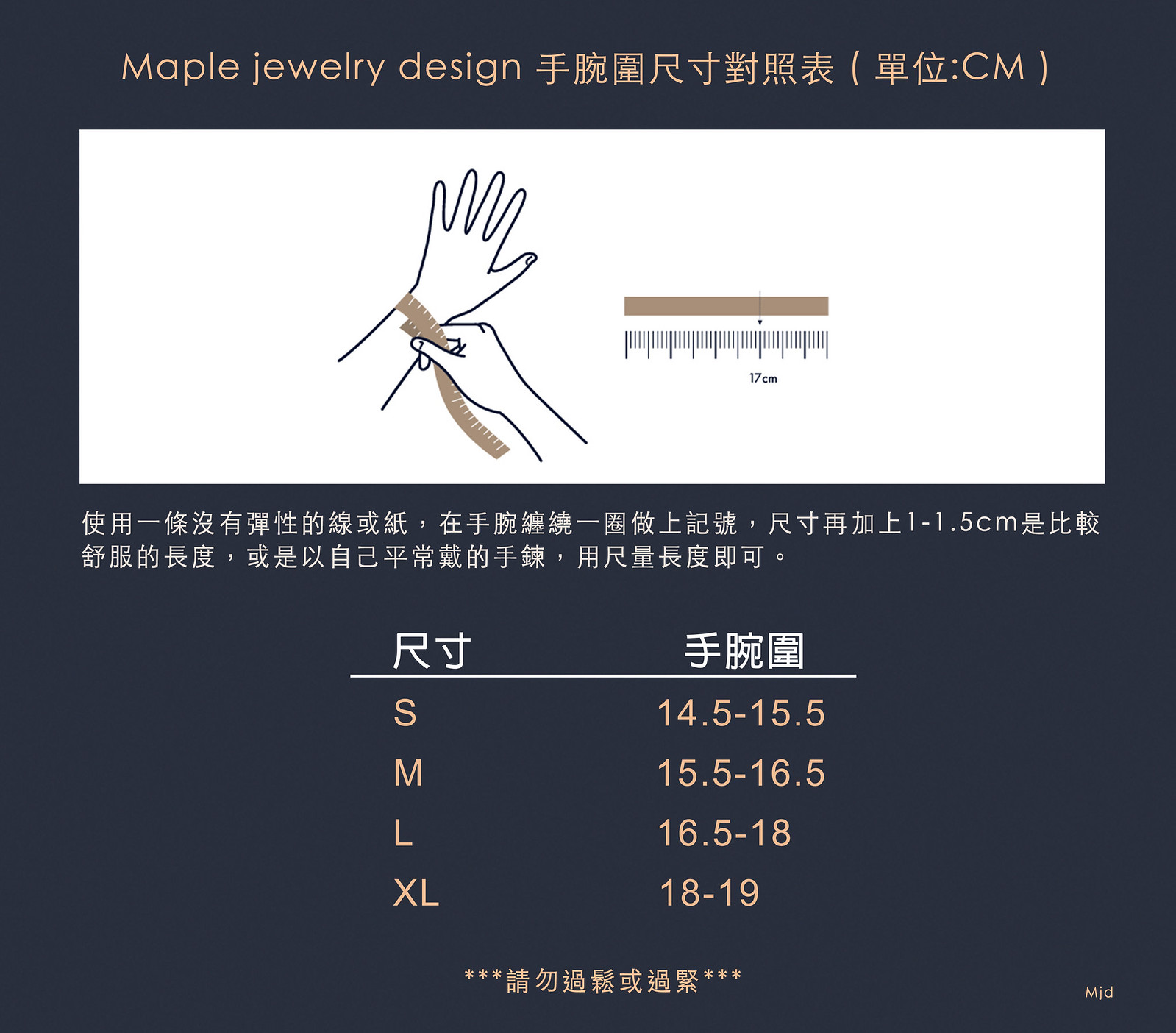This advertisement for Maple Jewelry Design features prominently at the top in a light mauve or pink font against a dark navy blue background. The text, "Maple Jewelry Design," is followed by a line of Asian glyph symbols, likely Chinese or Japanese. Below this, a horizontal white rectangle displays a black-and-white sketch of a woman's left hand, with her right hand wrapping a measuring tape around the wrist. To the right of this image is a scaled ruler or tape measure. Underneath the white rectangle, there are two additional lines of Asian text. Centered in the lower half of the image is a two-column table with larger Asian glyph symbols on the left and three glyph symbols on the right. Below a horizontal white line, the left column lists sizes: S, M, L, XL, corresponding to wrist measurements in centimeters (14.5–15.5, 15.5–16.5, 16.5–18, and 18–19 respectively) in the right column. The bottom of the advertisement features more Asian glyph symbols, flanked by three stars on either side. In the lower right corner, the small text "MJD" is barely discernible.